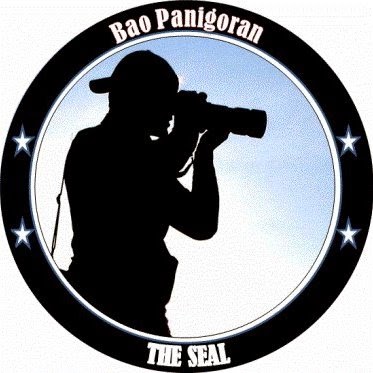The image features a circular logo with a predominantly black background and a minor white border. Encircling the logo is a black border bearing text in white: "Bao Panigoram" at the top and "the seal" at the bottom, both framed by two stars situated on either side. Centered within this black border is the dark silhouette of a man wearing a backward cap, intently peering through binoculars. The inner portion of the logo is occupied by this silhouette, which stands out against a predominantly white background. The overall aesthetic suggests a formal design, likely a company logo, as it resembles something you might find on a business card, a website, or perhaps even a pin. The colors used are primarily black, white, and light blue, ensuring a clean and professional appearance.